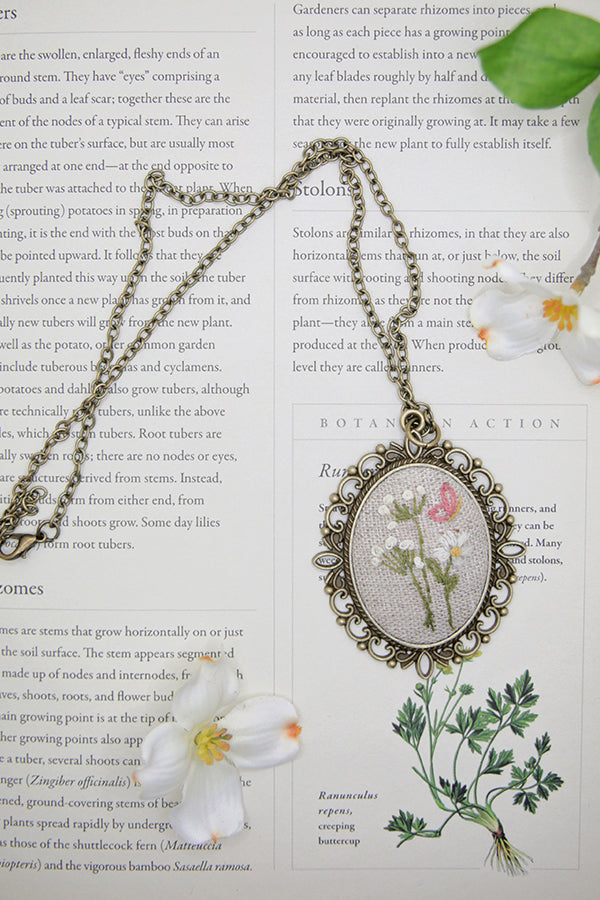The image is a vertically rectangular, full-color photograph of an open book or magazine page discussing botanical topics. The off-white page contains paragraphs of black text that mention "botany in action" and describe botanical features, including the "enlarged fleshy ends of a stem" with "nodes" and "leaf scars." There's also a botanical drawing labeled "Ranunculus repens, creeping buttercup." Laid across the page is a silver chain necklace featuring an oval-shaped pewter pendant. The pendant has a decorative border and contains a needlepoint-style design with white and pink flowers, as well as a pink butterfly. The upper right corner of the image showcases green leaves, while the center right displays a flower. In the lower right, a green plant with visible roots and leaves is present. Additionally, the page features two white flowers with yellow and orange accents. The scene is well-lit, suggesting the use of artificial light.